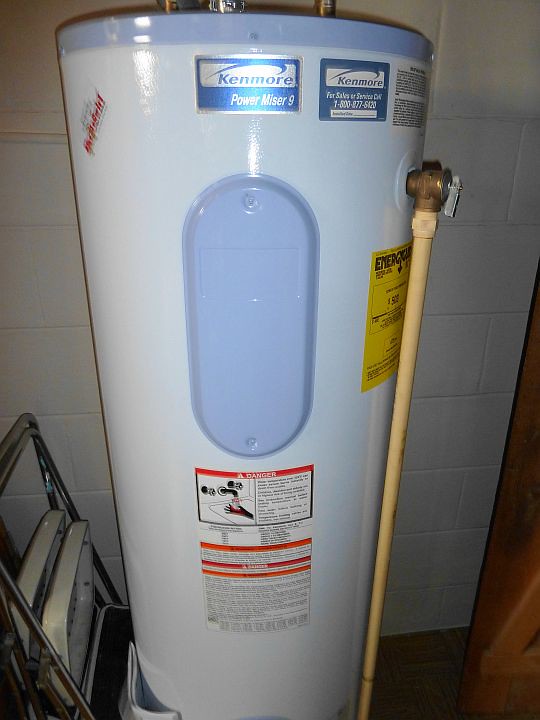This image depicts a Kenmore Power Miser 9 water heater, prominently displayed in a white brick-walled room that appears well-maintained, possibly a garage. The water heater stands tall and vertical with a primarily white exterior and blue accents on the front panel and top. It features several tags: a brand tag reading "Kenmore," and warnings including one illustrated with an image of someone getting burned by hot water. Additional warnings, in red and blue text, caution about hot surfaces.

The water heater includes an energy guide sticker on the right side and is marked with an ENERGY STAR label indicating potential savings of $500. Copper piping extends from the top and side, with the side pipe painted yellow as it descends. Adjacent to the water heater, on the left, is a small metal step ladder. The room itself is characterized by its fresh white-washed brick walls, suggesting recent refurbishment or a generally pristine condition.